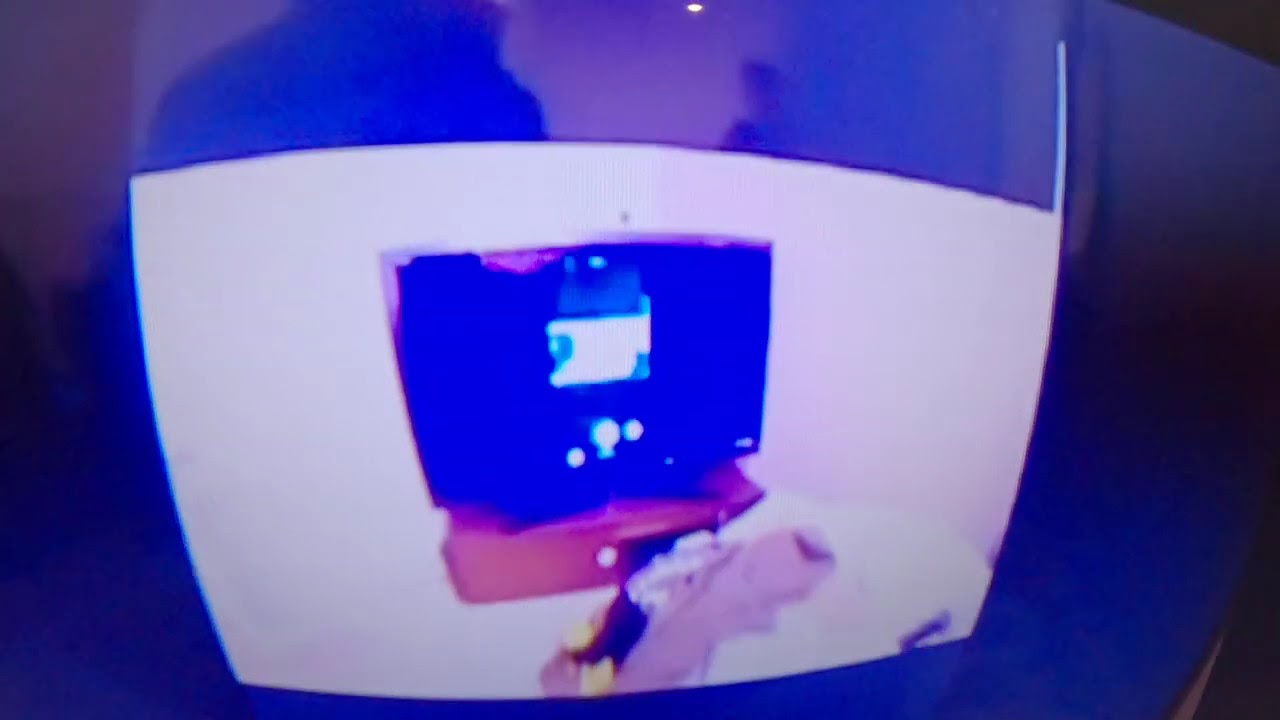This photograph features a television screen with a noticeable fisheye effect, making the image appear curved. The screen itself has a royal blue tint, suggesting the lighting within the room. On the television screen, there's a smaller black screen depicted, sitting on what looks like a red surface, possibly a table. To the bottom right of the main screen, there is a cartoon image of a dog. Shadows and reflections of the people taking the picture are visible on the screen, adding a layer of depth. The overall scene includes additional details such as a pink blanket, possibly with black clothing on it, and a pillow on the ground in front of the screen setup. The room, which appears to have white walls, adds to the slightly distorted and recursive appearance of the image, suggesting multiple layers of screens and reflections. The photograph is somewhat blurry, which adds to the complexity of discerning all the elements clearly.